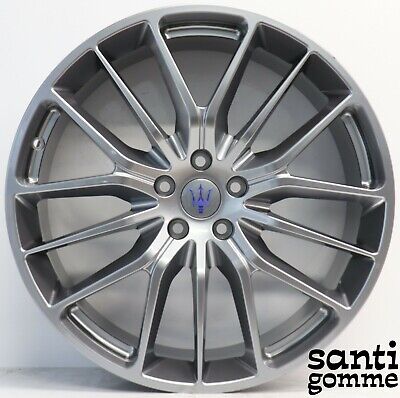In the image, a chrome or silver car rim is prominently displayed, leaning against a light gray-colored wall. The intricate design of the rim features 15 spokes arranged in five groups of three, radiating from the center, creating a star-like appearance. In the middle of the rim, there is a blue Maserati logo resembling a pitchfork, with lighter blue detailing, set against a perfect circular background. Surrounding this central emblem are five circular spots intended for lug nuts. Cast shadows are visible on the ground to the left side of the rim, adding depth to the image. In the bottom right corner, the text "Santee Gomee" is written in black lowercase letters. The wall in the background is primarily light gray on the top left and transitions to a whiter hue on the top right.